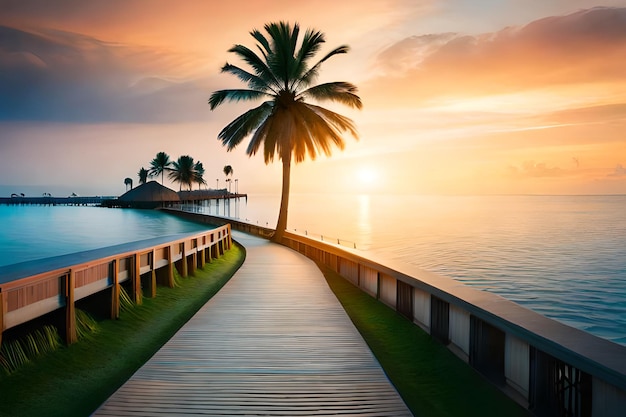The image depicts a serene tropical seascape at either sunrise or sunset, with a dazzling display of warm hues—pinks, yellows, and oranges—illuminating the sky and reflecting off the calm turquoise waters. A narrow, winding walkway bordered by railings extends through the scene, lined with lush green grass on both sides and leading toward the distant water. Dominating the center of the photo is a striking dark palm tree, adding a focal point to the tranquil scene. Farther along the walkway and in the background, the silhouettes of additional palm trees and some small cottages can be seen, casting shadows amidst heavy clouds. Ripples in the water catch the light, and the spherical sun hangs low in the sky, casting a white glow that blends seamlessly with the golden, peachy tones of the landscape.